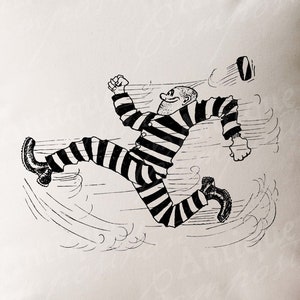A small, hand-drawn, black and white cartoon illustration shows a prisoner from an older era, identifiable by his traditional striped prison outfit. The prisoner, who may have very short hair or be bald, is caught in a dynamic running motion to the left, with his arms vigorously pumping—his left arm forward and right arm back. His exaggeratedly long legs add energy to his sprint, with short black lines emphasizing his high speed. Adding to the sense of urgency, his black and white striped beret has flown off and trails behind him to the right. His clenched fists and a determined expression on his face make it clear he's running away from something, most likely towards freedom. The entire scene, meticulously drawn in black ink on white paper, captures the essence of a rapid escape.